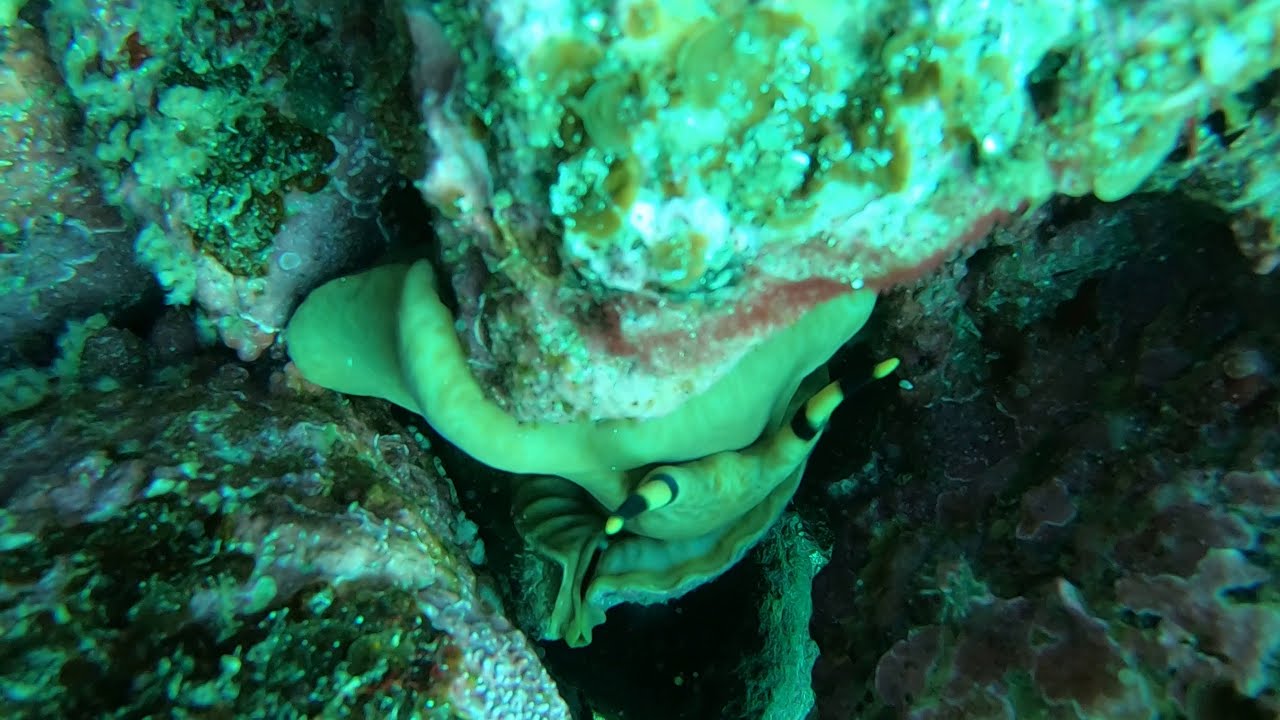This underwater photograph captures a mysterious sea creature suspended upside down from a rock. The creature is primarily light green, with distinct black and yellow stripes adorning its horn-like antennae. It blends seamlessly into its aquatic surroundings, making it difficult to identify. The rock itself is encrusted with white patches and a liberal coating of green algae. Surrounding the creature, several rocks display a rich palette of red, white, beige, and green hues, interspersed with blue moss-like patches. The water has a greenish tint, which deepens to a darker shade in the background, adding to the enigmatic and serene underwater scene.